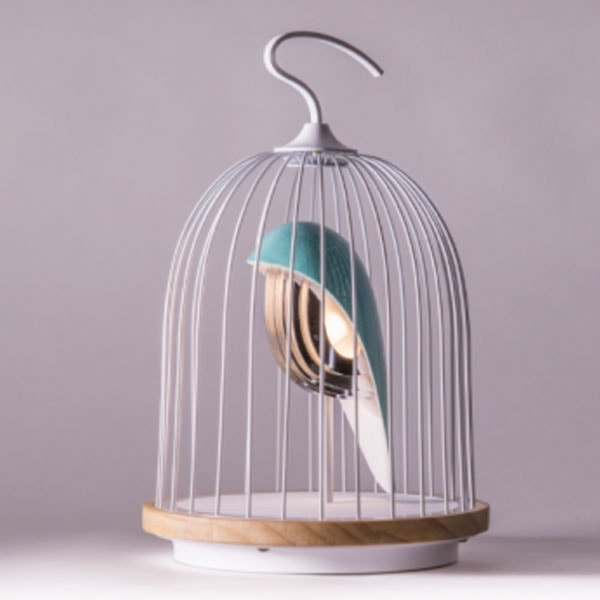This image depicts an ornate birdcage, primarily white and constructed from metal, with a wooden band encircling its pedestal base. The cage features vertical gray bars spaced about two inches apart, culminating in an elegant hook at the top for hanging. The backdrop is a gradient of gray, enhancing the detailed artistic display within the cage.

Inside lies an abstract, new-age sculpture reminiscent of a bird, though not a literal representation. This sculpture features a blue, scoop-shaped form that evokes a bird's body and tail, paired with five brownish-gold, semi-circular shapes suggesting a bird's breast or chest. The piece includes a small circular wing painted white, contributing to its dynamic, sculptural form. The absence of a head, legs, and beak emphasizes its abstract nature, making it a compelling piece of contemporary art.